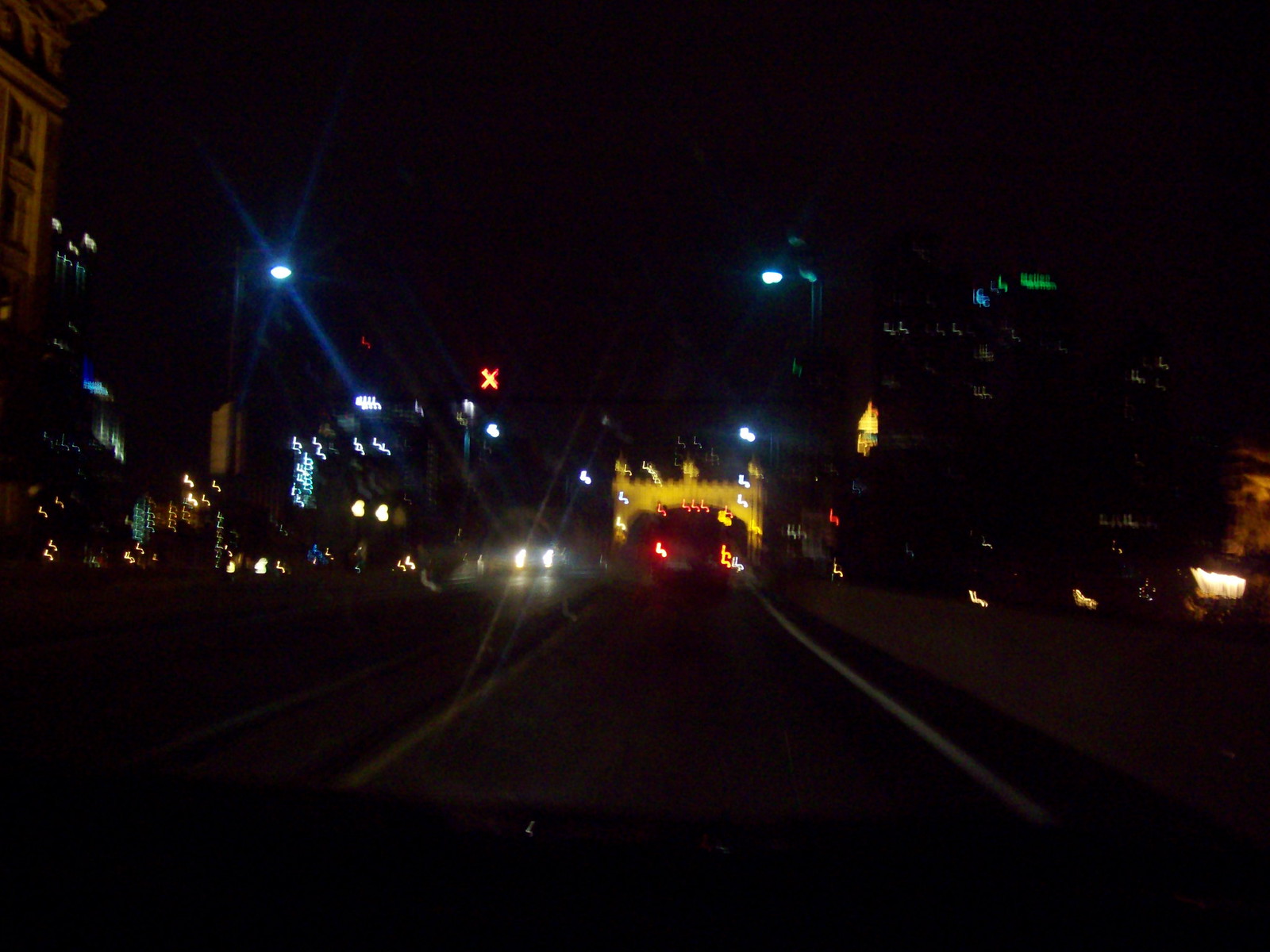A nighttime photograph, likely captured from either the driver’s or passenger’s seat of a car, showcases a dynamic cityscape. The road ahead unfolds beneath the city lights, steering towards a distinctive, yellow, bridge-like structure reminiscent of a castle. Just ahead in the same lane, a bus with glowing red taillights travels under this unique bridge. Simultaneously, a car with bright white headlights approaches from the opposite lane on the left side of the frame, adding a sense of movement and bustling activity. The backdrop is dominated by large office tower buildings, characteristic of a vibrant downtown core. The juxtaposition of the architectural scenery and the interplay of vehicle lights creates an evocative, urban night scene.